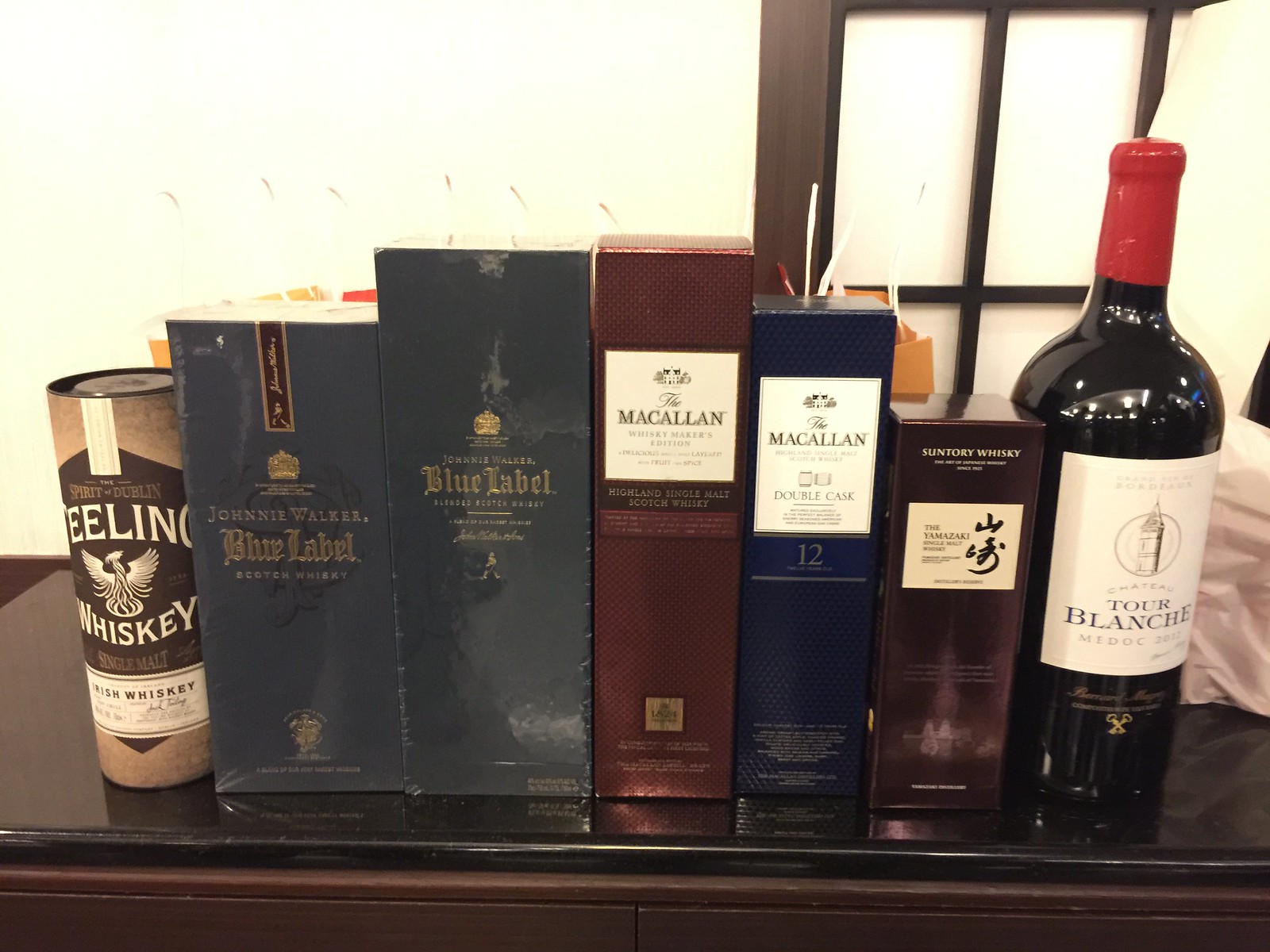The photograph captures a meticulously arranged display of various alcoholic beverages on a dark brown tabletop, set against a pale white background with a closed brown window frame to the right. Centrally positioned on the table, the arrangement begins on the far left with a cylindrical container labeled "Ealing Whiskey," primarily in shades of brown and light brown. Moving to the right, there are two thin green boxes both labeled "Johnny Walker Blue Label." Adjacent to these are two more boxes: one red and one green, both marked with "Macallan," with specific editions noted as "Double Cask" and "Whiskey Makers Edition" respectively. Further to the right, a shorter black box is inscribed with "Suntory Whiskey." On the far right of the display is a dark red bottle of wine, labeled "Tour Blanche," which is sealed with red plastic. The overall setting appears to be an indoor scene, highlighting a curated selection of fine whiskeys, scotches, and wine.